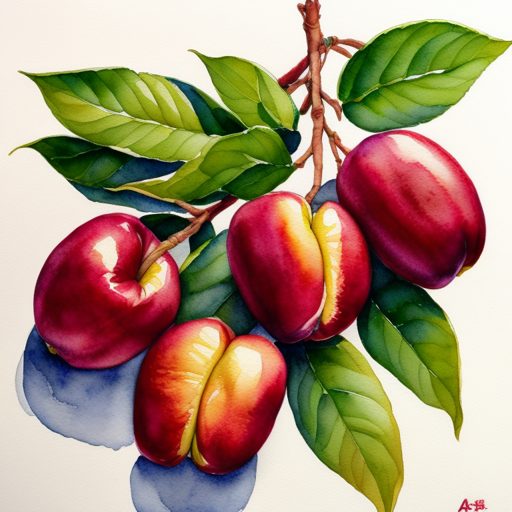The image depicts a square watercolor painting showcasing a branch adorned with four fruits that resemble peaches or plums. These fruits are primarily red with varying shades of yellow, particularly prominent in the center two, which have noticeable creases running from top to bottom, highlighting the yellow hues along these lines. The other two fruits have less pronounced creases but still exhibit some yellowing. The branch, emerging from the top center of the painting, extends with numerous sub-branches and lush green leaves that interweave with the fruits, creating a clustered, vibrant display. Below the branch on the lower-left side, there are bluish watercolor splotches adding depth and contrast to the painting. In the bottom right corner, a small inscription in red Japanese text, possibly the artist's signature, completes the scene.